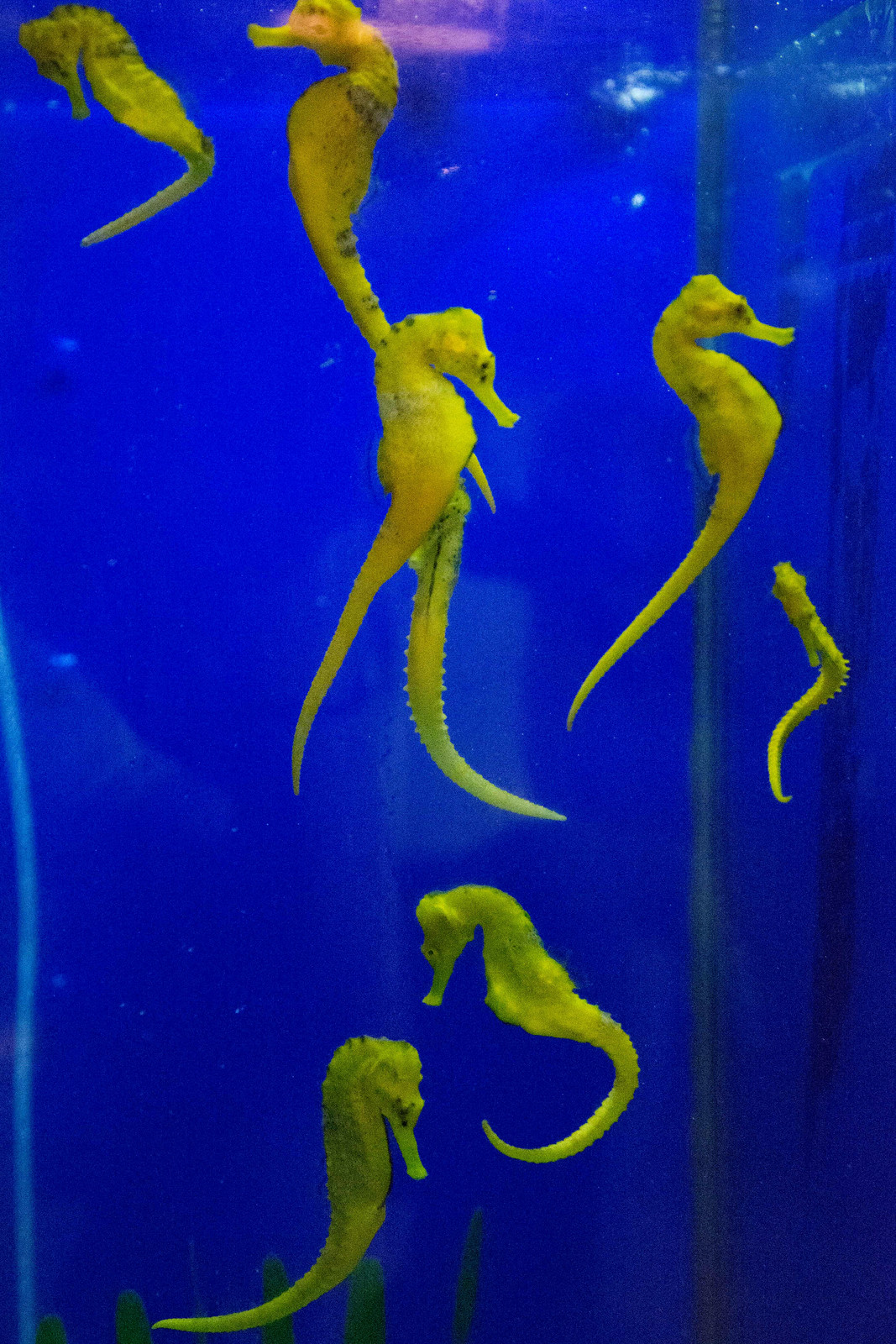The photograph captures a color image of a large aquatic tank filled with vibrant seahorses. The tank, which fills the entirety of the frame, features a deep blue background, perhaps due to the water or the glass itself. The water appears clear, hinting at its well-maintained environment. There are subtle reflections on the glass front, though their indistinct nature leaves their source ambiguous.

Dominating the scene are numerous seahorses, primarily yellow in hue, but displaying a range of tones from a rich egg yolk color to lighter shades with tinges of lime green. They are elegantly floating at various depths in the water, with many positioned in the foreground, providing clear side profiles. Their distinctive long snouts and curved tails are easily discernible, with some tails curling around their bodies while others extend freely. A particularly large seahorse occupies the center, notable for its exceptionally long tail, spanning nearly twice the length of its body.

In addition to the seahorses, a few green strands of seagrass can be seen near the bottom of the tank, adding to the naturalistic setting. Towards the top of the tank, small bubbles rise, enhancing the aquatic atmosphere. The black seal of the tank’s casing is faintly visible in the background. Overall, the image presents a captivating underwater scene, highlighted by the strikingly colored seahorses and their serene surroundings.